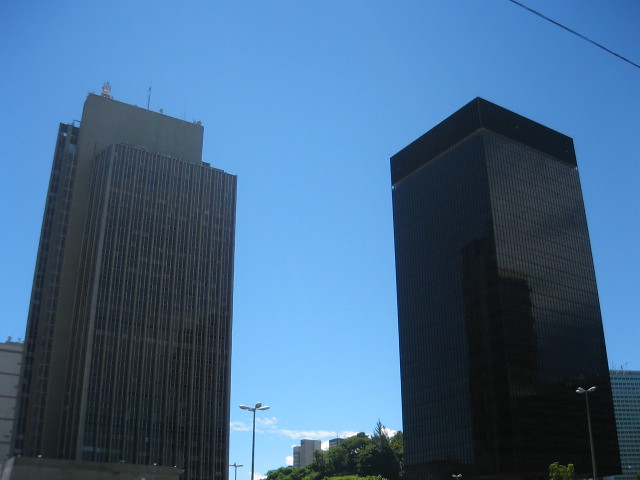This square image captures an upward view from street level, showcasing two opposing tall buildings against a clear blue sky with a few feathery white clouds scattered at the lower edge and distant background. The building on the left is brown with numerous windows, featuring a central divider resembling concrete. On the right, there is a black building, symmetrical in shape but differing slightly in detail, also adorned with many windows and a solid black top. Both buildings appear to be around 20 stories high and are likely business structures, situated in what seems to be an office park. Between them, at the bottom of the frame, light poles, green trees, and additional buildings can be seen, contributing to the urban scene. The clear sky, highlighted by minimal cloud coverage and space between the towers, amplifies the sense of vertical grandeur.